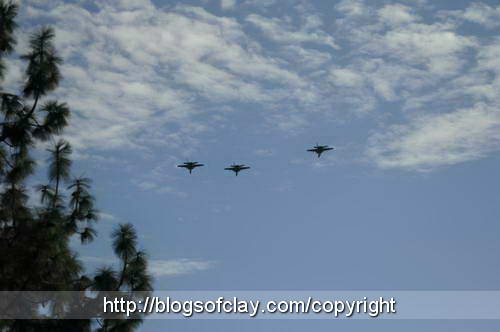In this photograph, we observe three military fighter jets flying in a loosely arranged semi-formation, heading away from the viewer. The aircraft are moving at a relatively slow speed, evident by their retractable swept wings positioned outward, not in their swept-back configuration. The jets are spaced with two closer together and a third further off to the right. The scene is set against a backdrop of a clear blue sky dotted with puffy white clouds. To the left of the image, there is an old-growth pine tree, adding depth and a touch of nature to the composition. Superimposed at the bottom of the image is a white text stamp: "http://blogsofclay.com/copyright."